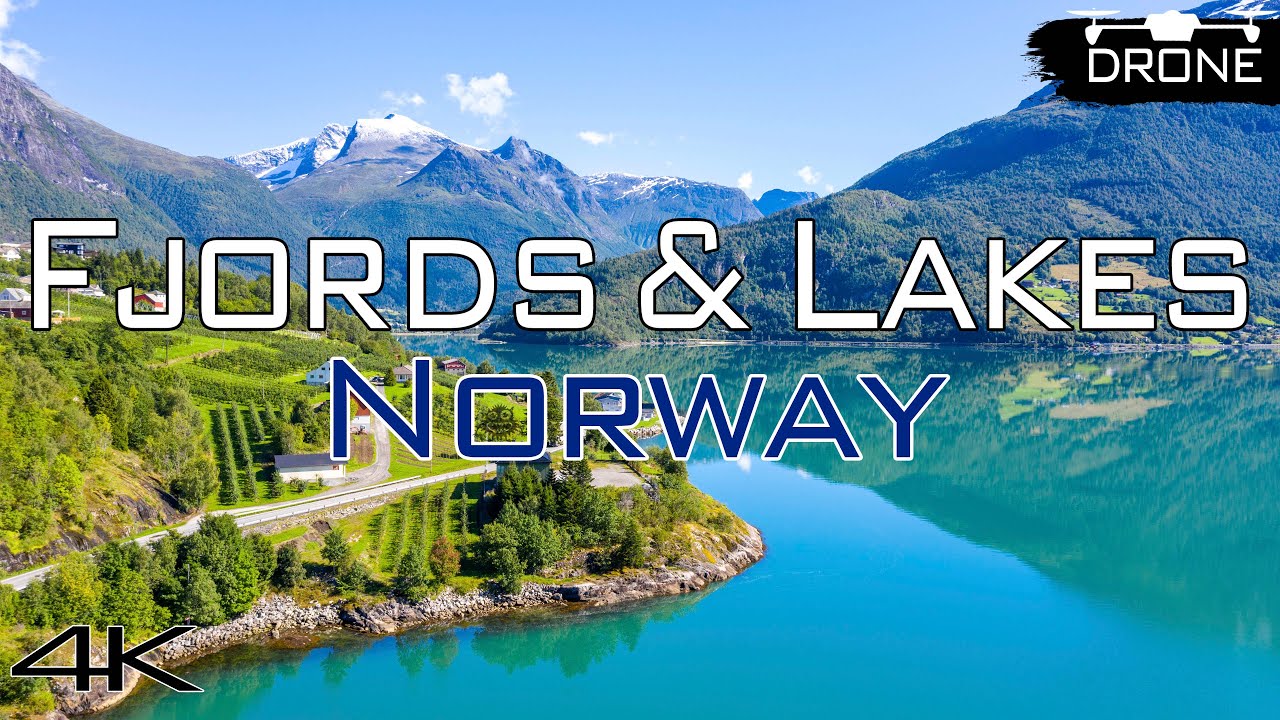The image is a vibrant rectangular photograph, used as a card, that seems to be from an advertisement or a title screen of a video, potentially showcasing shots captured by a drone. In the top right corner, there's a black splotch with the word "drone" written in white letters and an outline of a drone above it. Across the center of the image, in large white letters, it reads "Fjords and Lakes," and just below in dark blue letters with white edging, it says "Norway." The photograph showcases a stunning daytime view of a Norwegian landscape. 

The background features majestic snow-capped mountains under a bright blue sky scattered with small white clouds. At the center, there is a serene lake or fjord with mirror-like turquoise water that reflects the mountains above. From the left center to the bottom left, a lush, vibrant green peninsula extends into the water, covered with farmland, woodland, rows of trees, and crisscrossed by a road. Near the shoreline, rocks and dense green vegetation are visible. The scene appears serene and picturesque, making it an ideal showcase for the capabilities of a high-resolution camera, hinted at by the "4K" label in the bottom left corner.